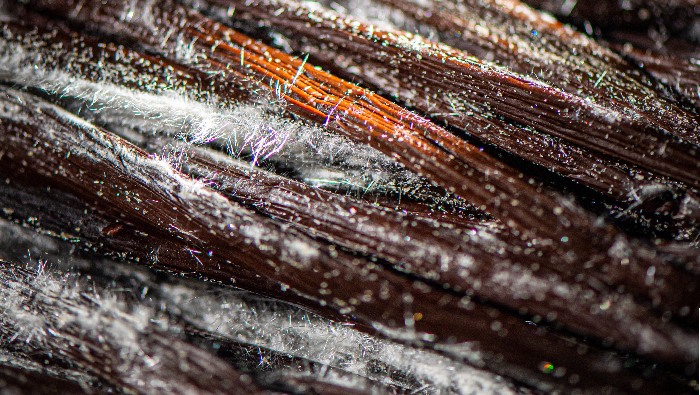This color photograph showcases an intricate array of thick, woody strands of an indeterminate material, stretching horizontally across a landscape of dark brown hues interspersed with lighter brown segments and patches of white. Some strands are enveloped in a delicate white substance, possibly indicating the presence of a fine particulate coating. Though the precise scale of the image remains ambiguous, there is a suggestion that it might be a microscopic view, adding an element of mystery to the composition. The dimensions of the image are wider than it is tall, with an absence of any identifiable text, people, animals, plants, flowers, trees, buildings, or motorized vehicles, which allows the viewer's focus to remain solely on the enigmatic material strands.